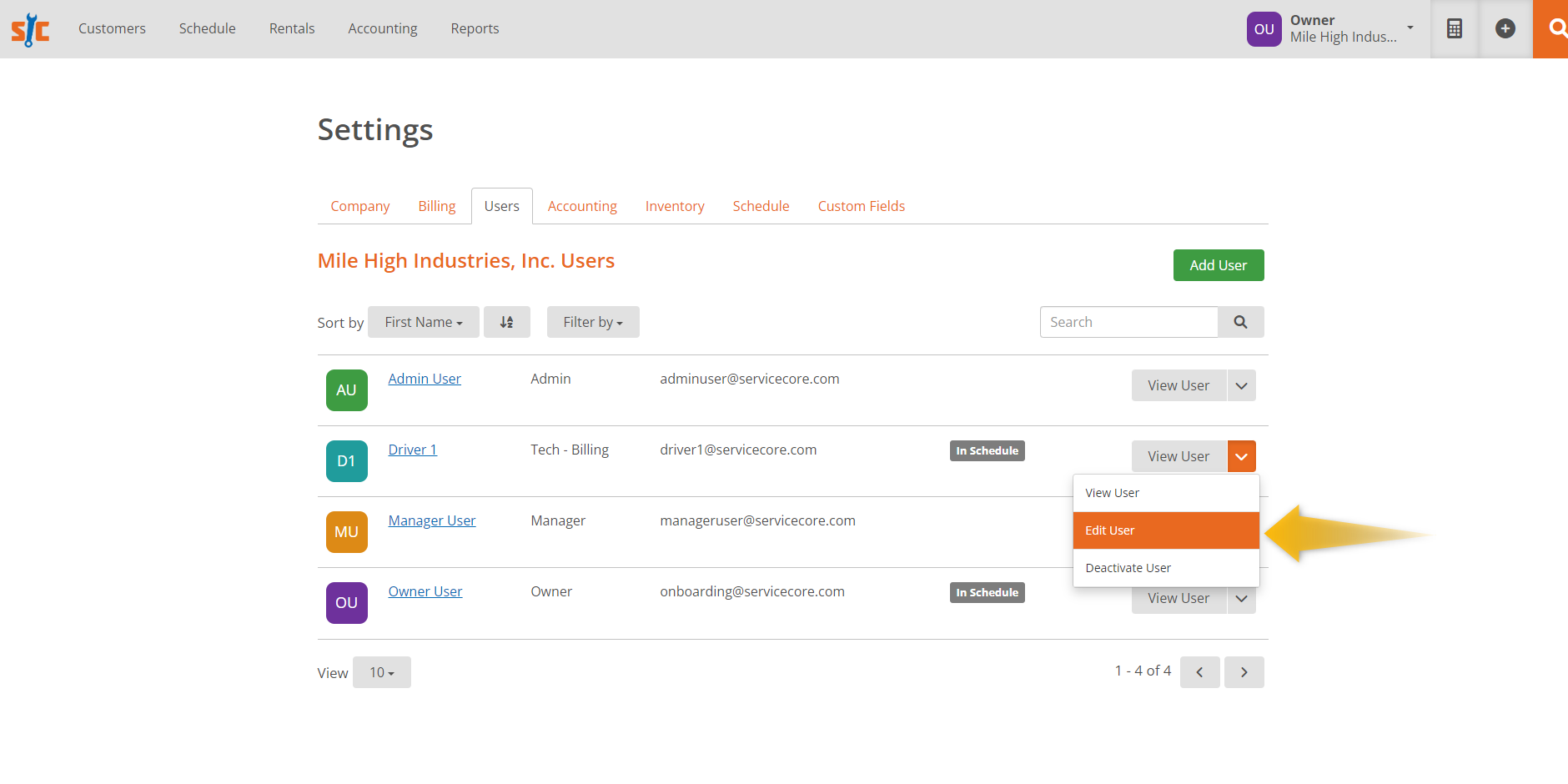The image depicts an airline membership user interface page. In the upper left corner, there's a logo featuring green and orange initials "SC" alongside a blue wrench icon. Nearby, several menu items are listed: "Customer," "Schedule," "Rentals," and "Accounting Reports." On the upper right side, there's the user profile section highlighted in purple displaying the initials "OU" and labeled "Owner, Mile High Industries," though it's abbreviated with "N-U-I-N-D-U-S" followed by an ellipsis. Adjacent to this are icons for sorting, adding, and searching.

The central area of the page is set against a white background with black text that reads "Settings." Beneath this, several categories are listed: "Company," "Billing," "Users" (which appears to be the selected category), "Accounting," "Inventory," "Schedule," and "Custom Fields." There's a dedicated section for "Mile High Industries Incorporated Users" with a green "Add User" button on the far right.

Below, the interface allows sorting users by first name, accompanied by a "Filter By" button. Various user roles are displayed: 
- "Admin User" as Admin.
- "Driver One" with the role of Tech Billing.
- "Manager User" as Manager.
- "Owner User" as Owner.